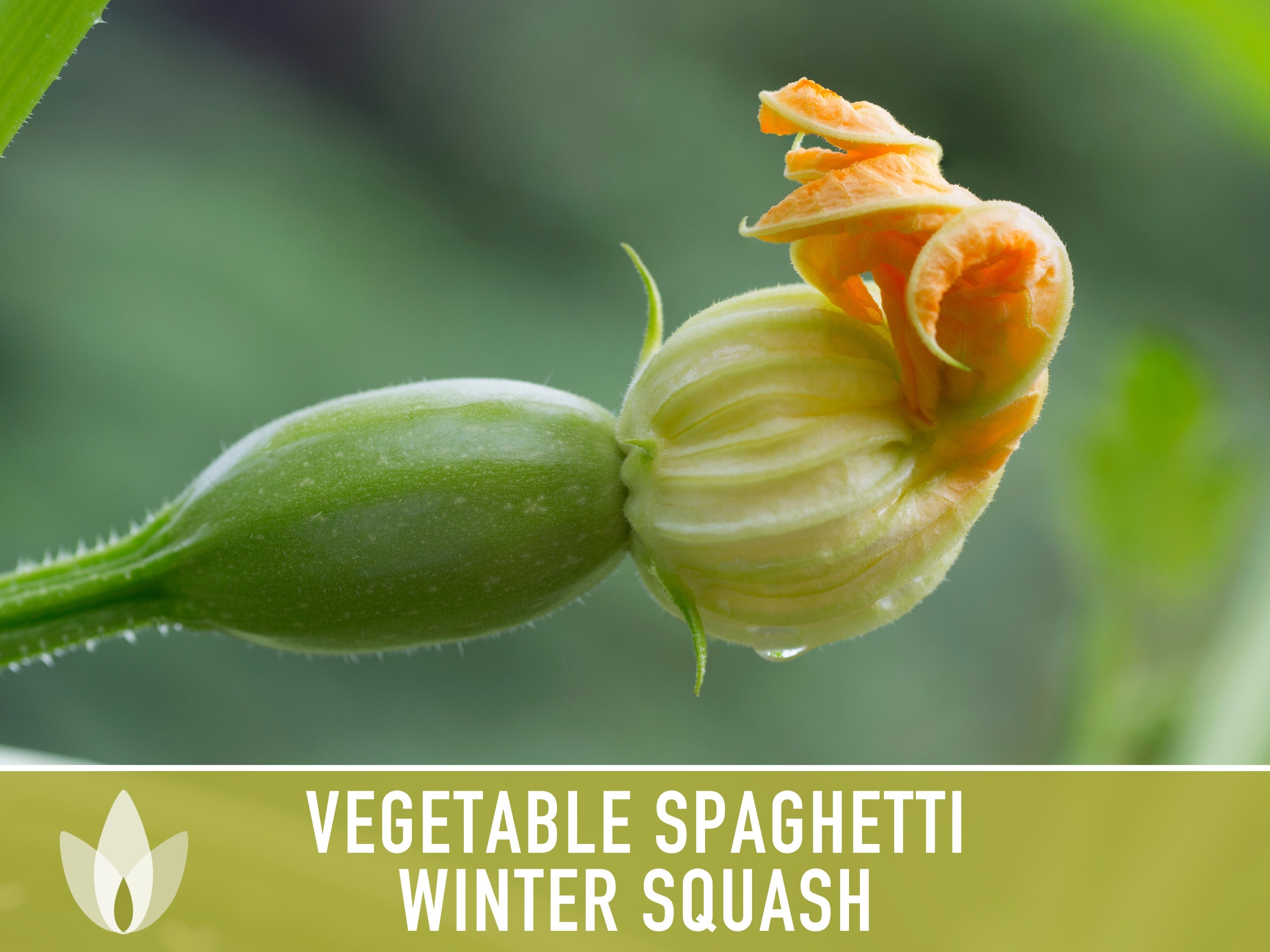The image is a highly detailed, close-up photograph of a vegetable spaghetti winter squash emerging from a green stem. The squash itself is prominently orange with white-tipped curls, signaling the early stages of its growth. The stem is deep green and covered with fine cilia, hinting at its developing stage. The background is blurred, likely depicting a garden area, but it remains indistinct. The photograph appears to be part of an informational card: the bottom quarter features a solid olive green bar with the text "vegetable spaghetti winter squash" next to a foliage flower logo. The vibrant orange and green hues of the squash contrast strikingly against the softer backdrop, emphasizing the intricate details of the plant as it begins to flourish.